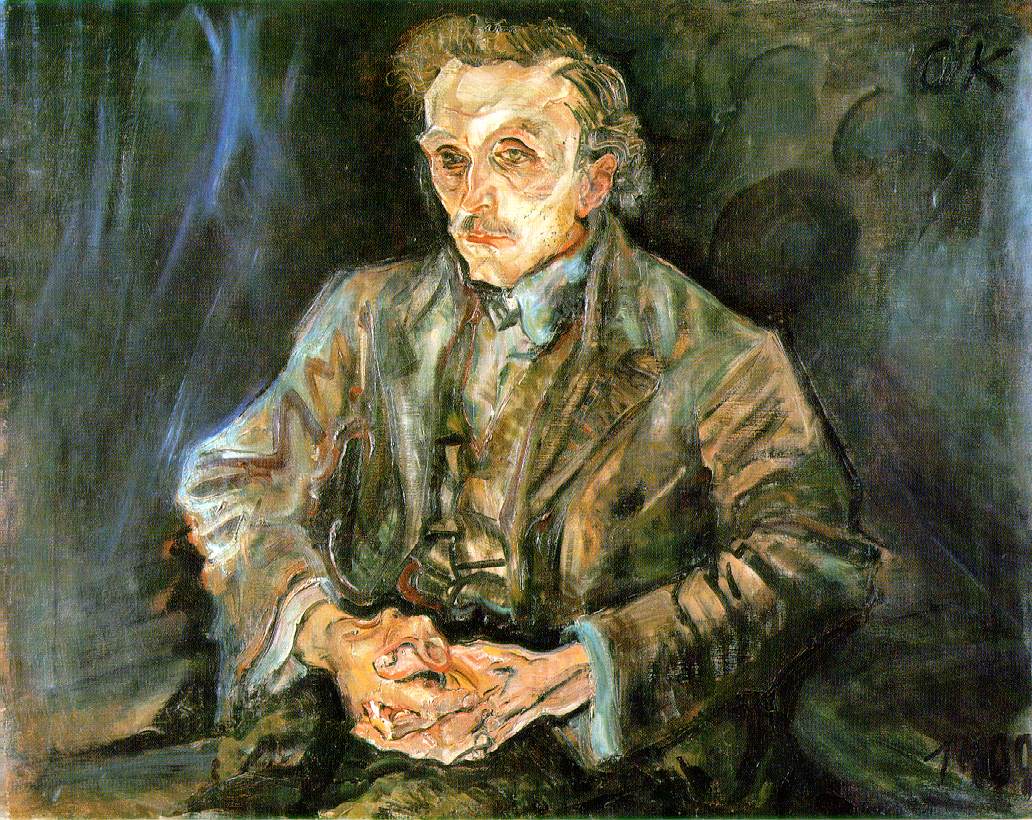This painting features an elderly man, likely in his 60s or 70s, presenting a somber and contemplative demeanor. He is seated facing forward, arms folded on his lap. The man, who bears a resemblance to a young Albert Einstein, has a mustache and disheveled grayish-brown hair. He dons a dark, likely black or very dark brown, wrinkled suit jacket over a white, ruffled shirt, and his pale skin suggests he is Caucasian. The background of the painting is dark, dominated by hues of black, gray, and dark green, creating a muted, smoky ambiance. A light blue streak on the left side and assorted shapes hint at an abstract, old-style artistic approach. On the lower right side, an unreadable signature is visible. The overall use of brush strokes and the simulated light source adds depth and texture to the scene, portraying a thoughtful yet serious atmosphere.